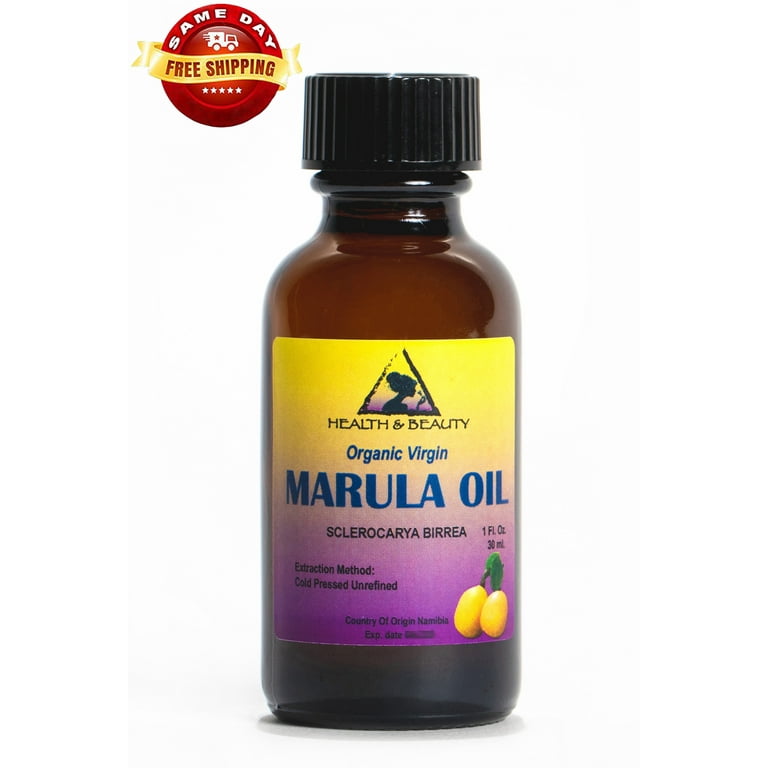This product photo showcases a small, brown glass bottle of organic virgin marula oil, prominently labeled with "Health and Beauty." The branding includes a triangular logo featuring a silhouette of a lady. The label displays a vertical yellow-to-purple ombre design and lists the scientific name Sclerocarya birrea, indicating the marula oil is cold pressed and unrefined. The bottle contains one fluid ounce (30 milliliters) and is sourced from Namibia. The bottom of the label features an illustration of two yellow fruits, likely representing the marula fruit, and the bottle is topped with a black cap. An expiration date is present but blurred. Additionally, a digital banner in the top left corner of the image announces "Same Day Free Shipping" in red and yellow text.